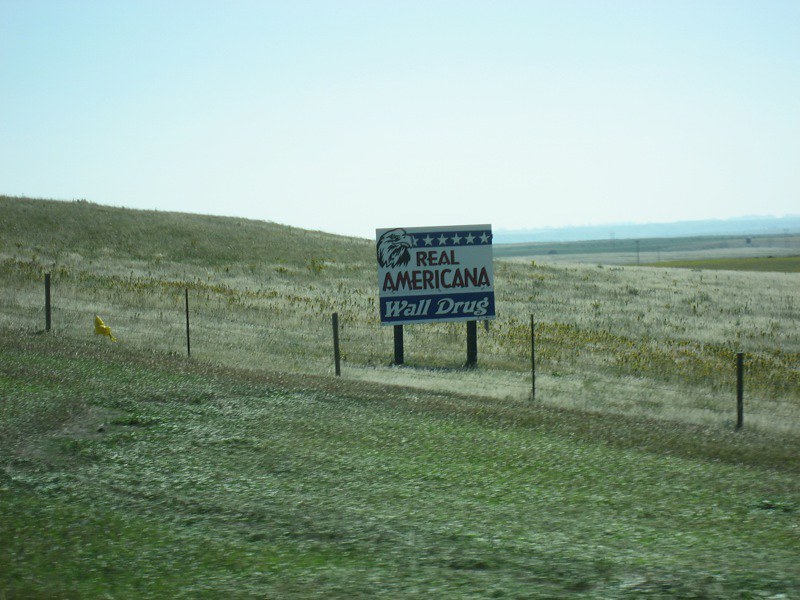A large sign stands prominently in an open field, not far off the ground. The sign reads "Real Americana Wall Drug" in blue lettering on a white background. At the top, an image of an eagle is prominently featured. The upper border of the sign includes a blue strip adorned with white stars, while the bottom has a blue strip with white writing. The sign is positioned within a wire-fenced area, inside of which there is a mysterious yellow object that appears pointy and round. The surrounding landscape is predominantly green grass, particularly lush on the side closest to the camera. The expanse of the field stretches endlessly into the distance, culminating in a tree line that marks the horizon. The image captures the vast, open space typical of rural Americana.